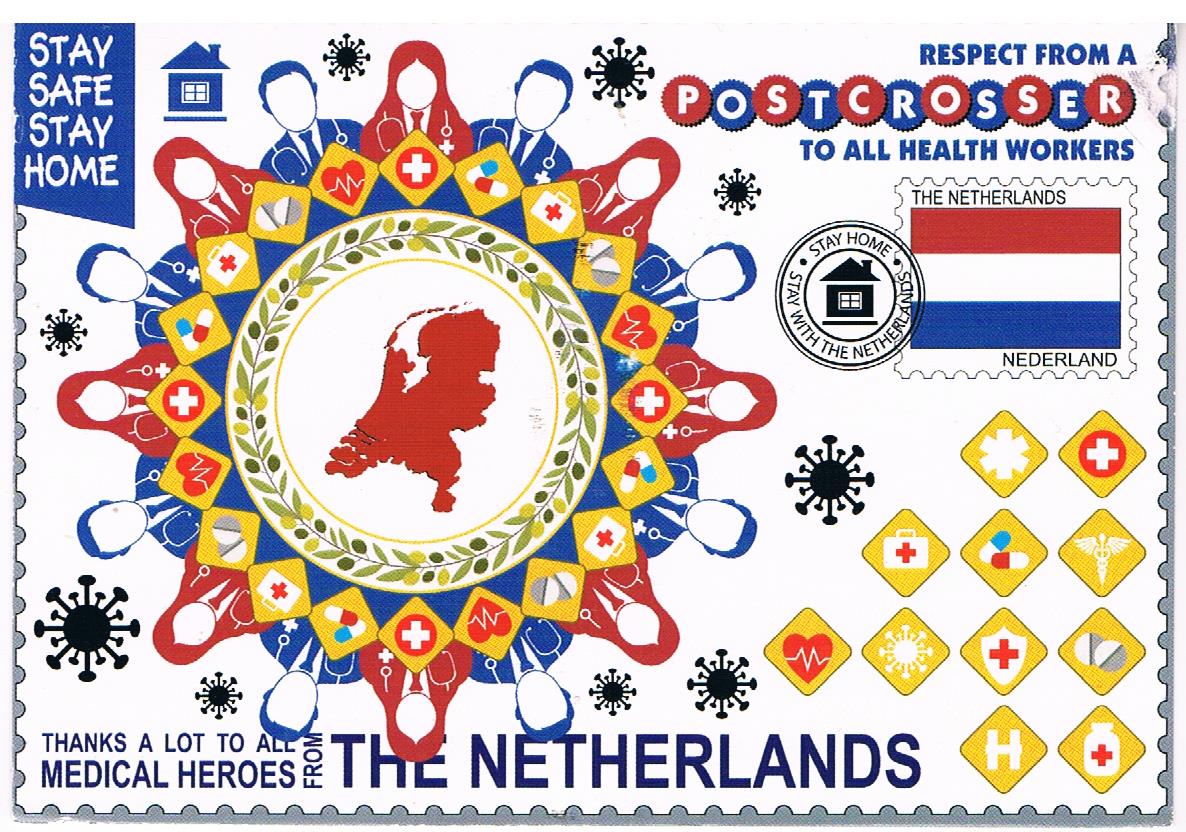This image features a rectangular stamp with a predominantly white background. In the upper left corner, a blue box with white text reads, "Stay Safe, Stay Home," accompanied by a small blue house graphic. To the right, bold text in alternating red and blue circles states, "Respect from a Post Crosser to All Health Workers." Below this, a circle encloses illustrations of medical personnel—men in blue and women in red—encircling a central motif of green olive leaves and what appears to be a map of the Netherlands. Scattered around this central circle are icons representing medical themes, including a red heart with a heartbeat line, medical kits, pills, and red crosses. At the bottom of the stamp, the text, "Thanks a lot to all medical heroes from the Netherlands," emphasizes the tribute’s intent.